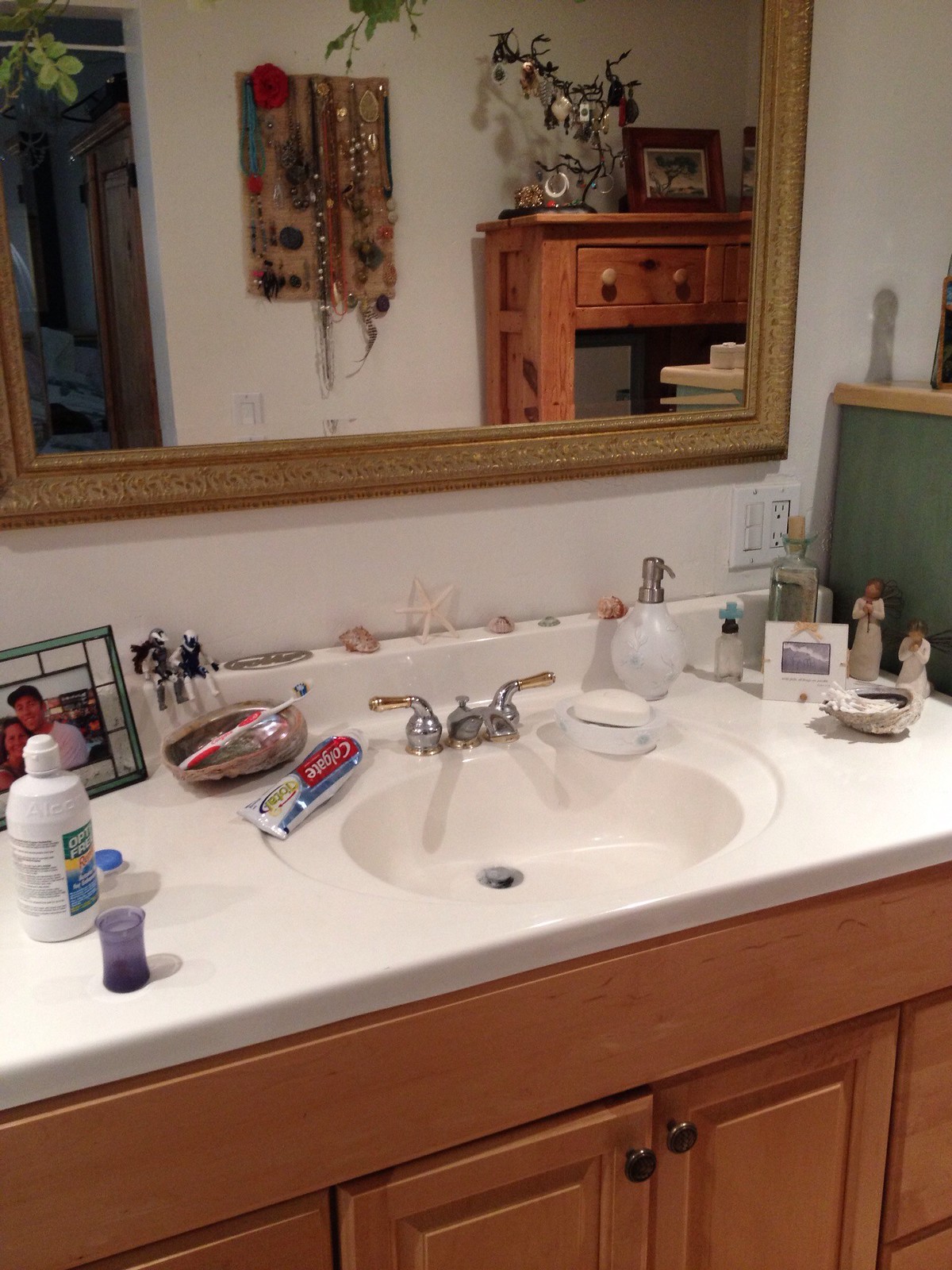This color photograph captures a section of a bathroom with notable clarity and detail. The focal point is a pristine white sink situated on a matching white countertop. Below this, a cabinet made of medium-toned wood adds a warm, pleasant contrast to the predominantly white fixtures. Mounted above the sink is an expansive mirror that reflects the room's opposite side, revealing a large chest of drawers in a complementary medium brown wood. Atop this chest sits a framed photograph along with a miniature silver object resembling a Christmas tree.

On the countertop to the left of the sink, a Colgate toothpaste tube lies beside a white bottle, likely of lotion, though the label is indiscernible. On the right side of the sink, a white soap dish holds a substantial white bar of soap. Nearby stands a tall, white bottle with a silver dispenser top, accompanied by a couple of other light beige bottles, likely containing personal care products. This detailed setup evokes a sense of cleanliness and organization within the cozy space.